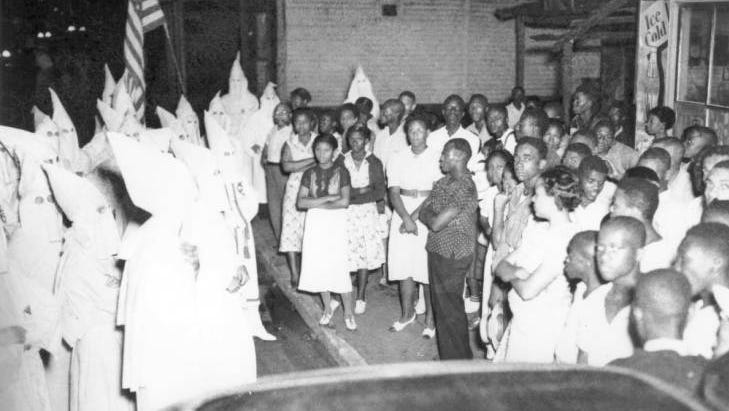This detailed, black-and-white photograph, likely from the 1940s or 1950s, portrays a tense civil rights standoff. On the left side, a dozen or so members of the Ku Klux Klan stand together, adorned in their notorious white, ghostly robes and hooded attire with eye slits, set against a dark, possibly nighttime backdrop. The Klansmen are bunched up and standing resolutely. On the right side, facing them, is a group of African American individuals, comprising both adults and children, standing in silent opposition. The gathering appears to be situated in front of a storefront, with an American flag visible in the background and a banner that reads "Ice Cold." The photograph, grainy and faded, evokes a palpable sense of confrontation and highlights the era's racial tensions.